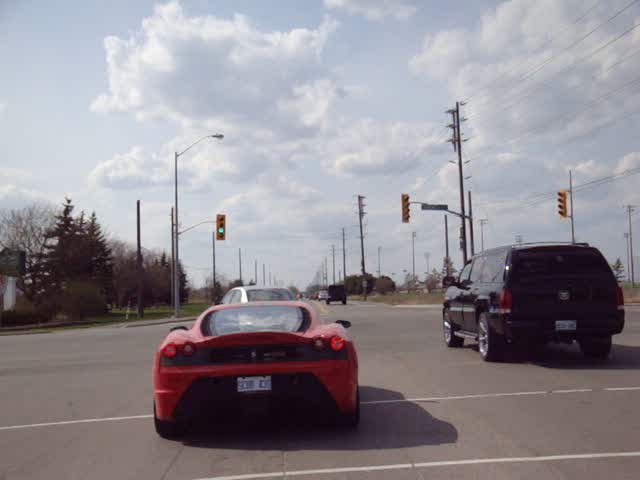This image captures a busy city intersection under a cloudy sky, characterized by billowy, puffy clouds. In the forefront, a gray car is positioned within the intersection, with a striking red sports car, possibly a Lamborghini or a Ferrari with a white license plate and black trim, right behind it in the left-turn lane. To the right of the sports car, in the adjacent lane, there's a long black SUV with chrome rims, potentially a Cadillac, heading straight. The stoplights suspended above the intersection show one green light. The scene includes a variety of surrounding elements: to the left, a row of evergreen trees lines the roadside, while to the right, streetlights stand adjacent to a grassy verge which is bordered by a row of power lines. The road surface is blacktop, and the crosswalk is marked by two straight white lines. The photograph, seemingly taken from a vantage point in front of another vehicle, provides a clear, unobstructed view of the intersection ahead, giving a comprehensive look at urban traffic and infrastructure.